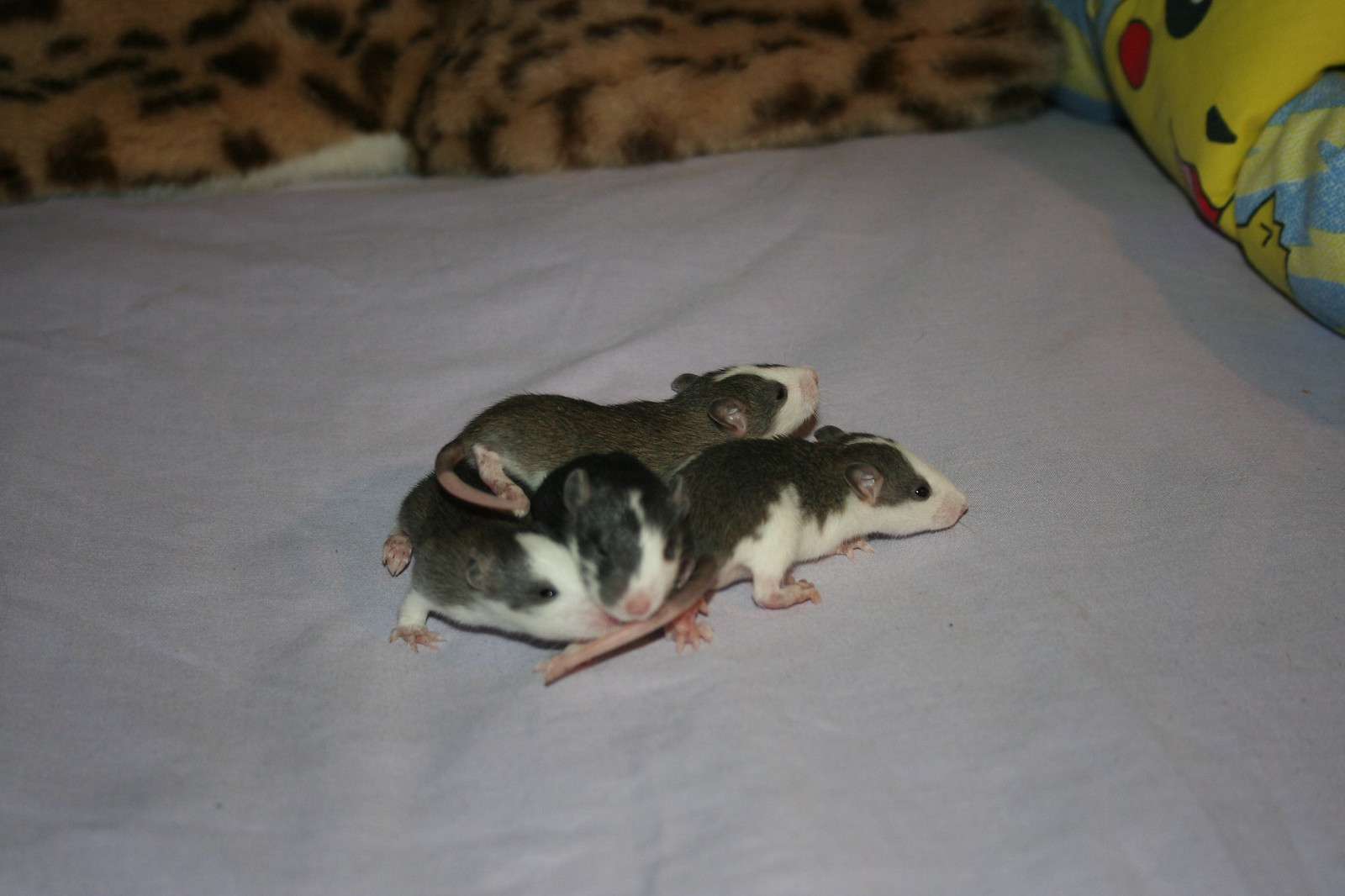The image depicts a close-up color photograph of four baby rodents, likely mice, lying together in a pile on what seems to be a bluish purple, possibly gray, sheet or pillowcase. These tiny creatures are nestled together, some overlapping, likely for warmth. They exhibit distinct physical features: pink noses, pink paws, long pink hairless tails, and small black beady eyes. Their fur is a stark contrast, with white underbellies, faces, and dark-colored fur on their backs that ranges from black to shades of brown or gray. Some have pink accents in their tiny ears. The background features a vibrant setting with a leopard print blanket, a beige and brown cheetah print fur pillow or blanket, and a yellow item showcasing Pikachu's face from Pokemon, distinguished by its black eyes, red blush marks, and a red mouth. This detailed scene highlights the tender and adorable appearance of the baby rodents amid a colorful, childlike surrounding.